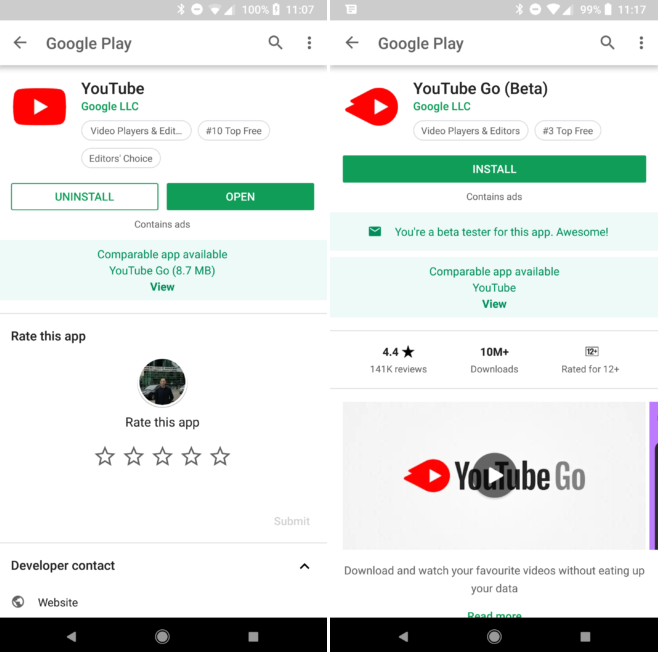The image showcases two screenshots of a smartphone displaying the Google Play Store. On the left screenshot, the user is browsing for the standard "YouTube" app, while on the right screenshot, the user is viewing the "YouTube Go" app, which is indicated to be in beta. Both screenshots highlight the user’s full battery at 100%. The timestamps on the phone show 11:07 AM on the left and 11:17 AM on the right, suggesting the screenshots were taken ten minutes apart as the user potentially evaluates the two YouTube app options. The contrasting interface details and app descriptions may help the user decide which version better suits their needs.